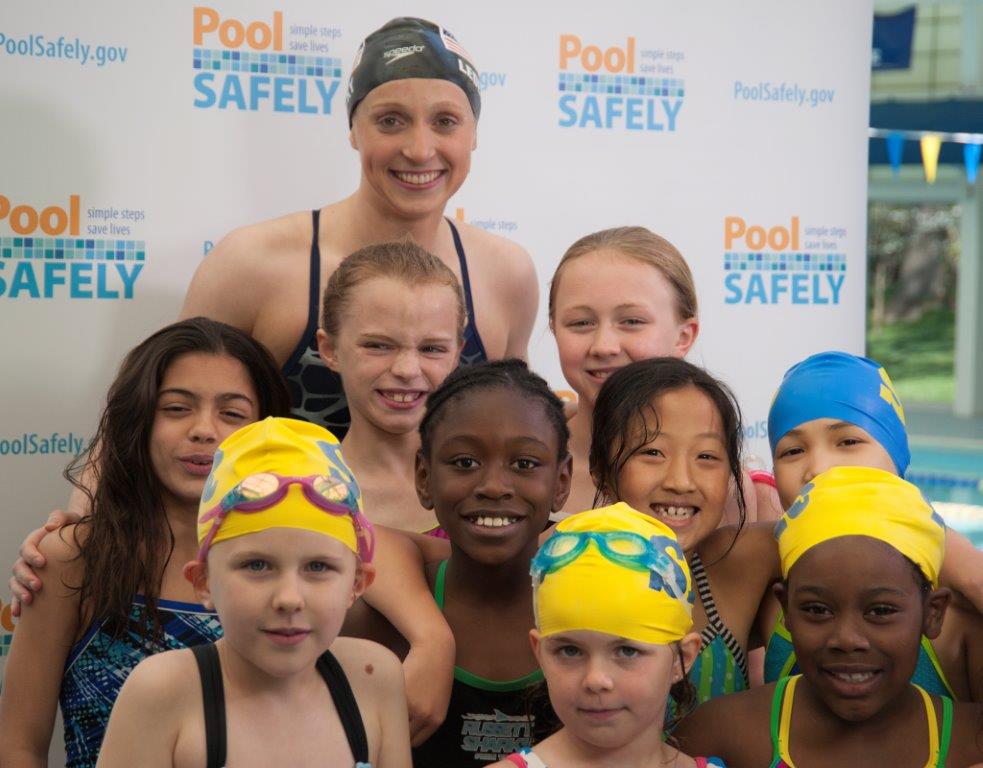In this vibrant and diverse outdoor photograph, a confident woman stands at the center of a group, embodying leadership and safety in swim instruction. She is a white female, clad in a black swimsuit with a white design on the front, and a black swim cap. Surrounding her are nine children, representing a beautiful mix of races and ethnicities, all wearing swim gear, signifying the inclusive nature of the event. 

To the left, a little dark-skinned girl with long brown hair stands near the forefront, alongside a white boy with orange hair, donning a yellow swim cap. An African-American child is centrally placed, beaming at the camera, and nearby, another African-American girl sports a yellow swim cap. An Asian girl, also smiling, adds to the diversity of the group. There's another small child in a swim cap, somewhat smiling, alongside a girl in a blue cap partially blocked from view. These children range in age from approximately six to ten years old.

Behind them, a sign emphasizes the theme of the day: "Pool Safety" and "PoolSafety.gov," in bold orange and blue hues against a white backdrop, suggesting a professionally organized event focused on promoting swimming safety. The colors in the image include various shades of blue, yellow, purple, orange, peach, black, brown, and white, creating a cheerful and unified presentation.